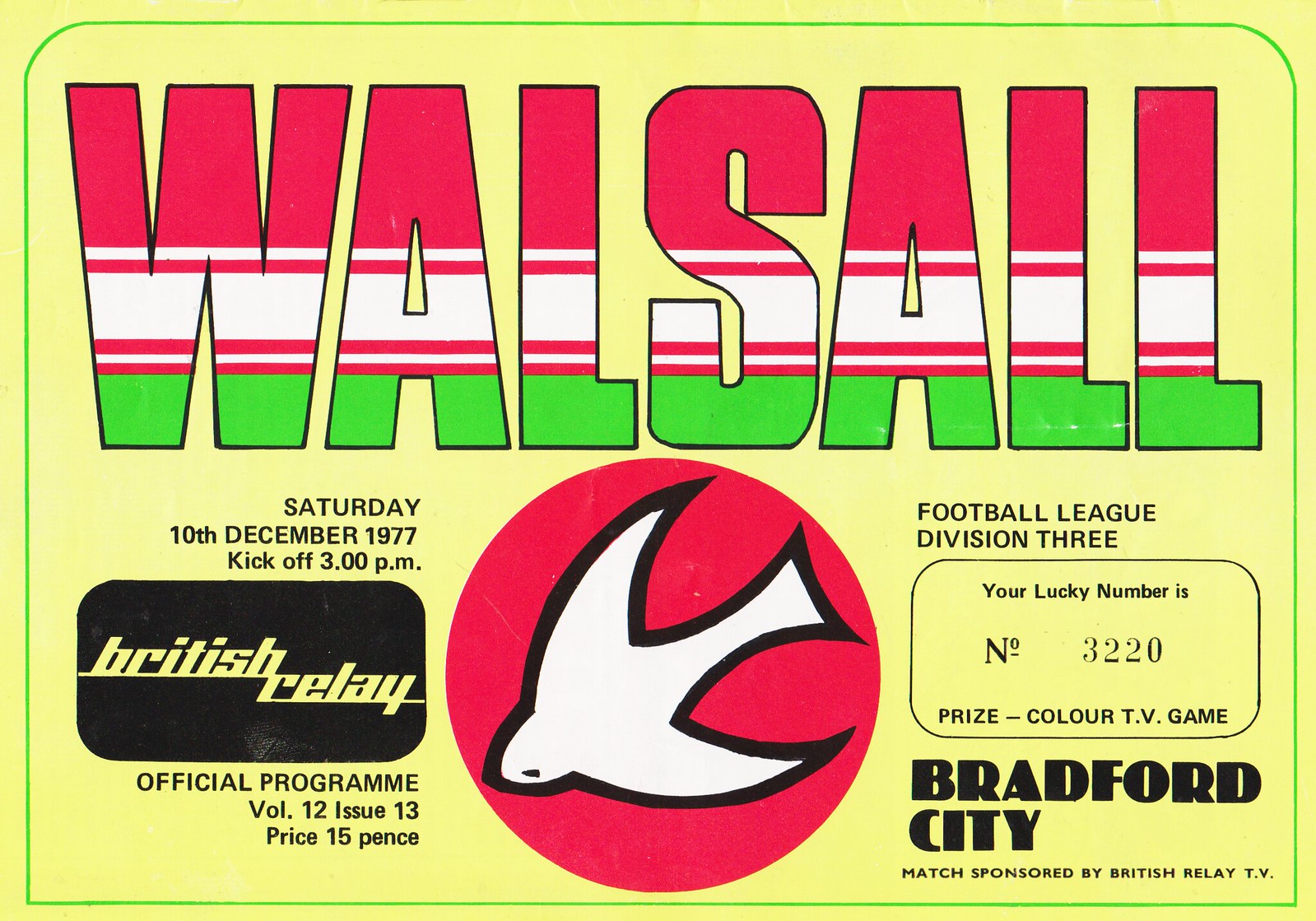The image displays a vibrant advertisement set against a yellow background, bordered by a thin blue line. Dominating the top portion of the image are large, bold letters in multicolored fonts (red, white, and green) spelling out "Walsall" (W-A-L-S-A-L-L). To the left, there is a rounded black rectangle with the italicized yellow text "British Relay," resembling a logo. Above this, in smaller black text, the date and time "Saturday, 10th December 1977, kickoff 3 p.m." are displayed.

Below, in black text, it states "Official Program, Volume 12, Issue 13," followed by the price, "15 pence." In the center at the bottom of the image, a striking red circle contains a white dove with a black outline. To the right of this emblem, additional details include "Football League, Division Three," your lucky number "3220," and the prize "Color TV Game." At the bottom right, bold black text spells out "Bradford City." The entire piece is marked by its clear and colorful design, indicating it is a program sponsored by British Relay TV.